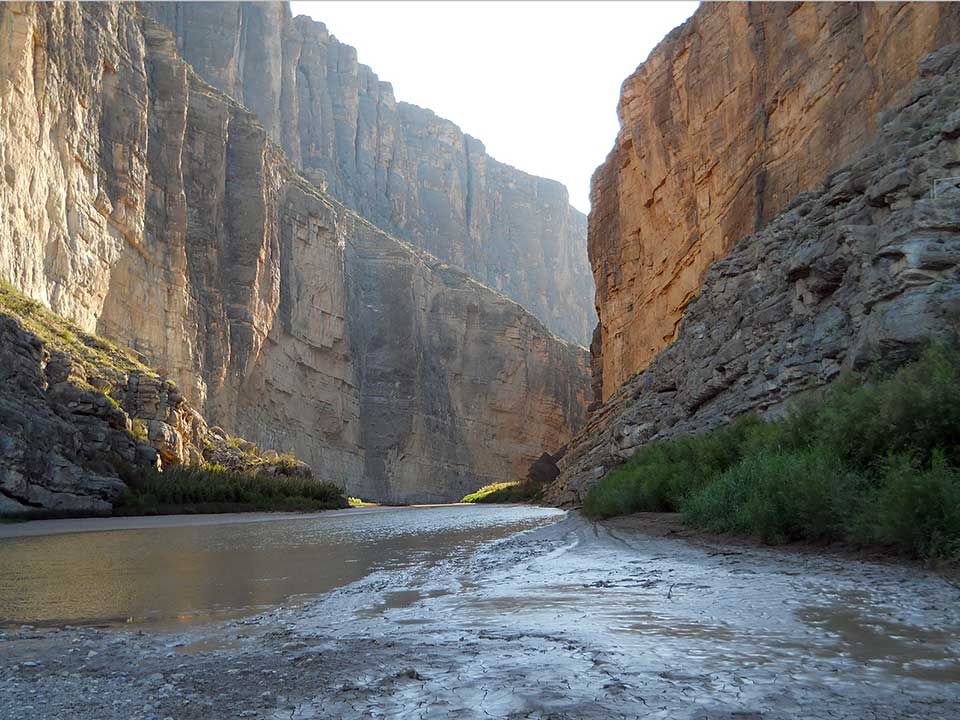This photograph captures a narrow stream coursing through a deep, rocky canyon. The stream, originating from the left and flowing toward the back central area, is lined with green bushes on both sides. The water itself appears gray and murky, with subtle ripples suggesting a steady but calm flow. In the bottom right corner, the streambed transitions into dry, cracked mud, hinting at the interplay between water and dirt.

The towering rock formations, which rise prominently on either side, are layered from millennia of sedimentation. These imposing structures have mostly straight edges, giving the illusion of walls rather than traditional peaked mountains. The varied colors of the rocks—stone, brown, and white—contrast with the greenery below. The sky can be seen at the very top of the image, although it's indistinct and white due to the brightness. The overall scene is bright and sunlit, leaving the sky featureless but illuminating the rich textures and layers of both the rocks and the vibrant vegetation.